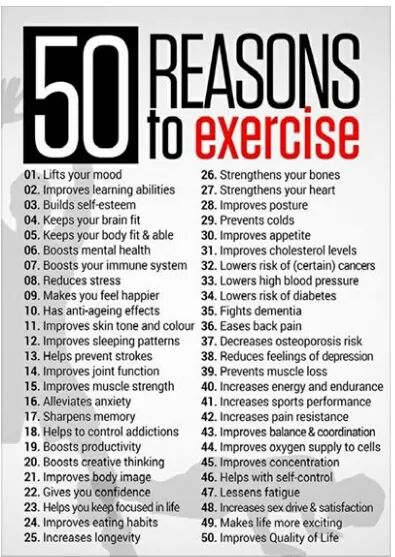This illustrative poster on a gray background promotes the benefits of exercise with the title "50 Reasons to Exercise" prominently displayed. At the top, a black box with large white text marks "50," followed by "Reasons" in black and "to Exercise" in red, creating a striking visual contrast. The background features dark gray silhouettes of two people working out: one standing with hands raised on the left, and another doing push-ups on the lower right. The list of reasons is displayed in two columns, starting with "1. Lifts your mood" and including benefits like "2. Improves learning abilities," "3. Builds self-esteem," "4. Keeps your brain fit," and "5. Keeps your body fit and able," continuing down to "50. Improves quality of life." The overall design uniquely combines illustration with graphic elements to effectively convey the message.